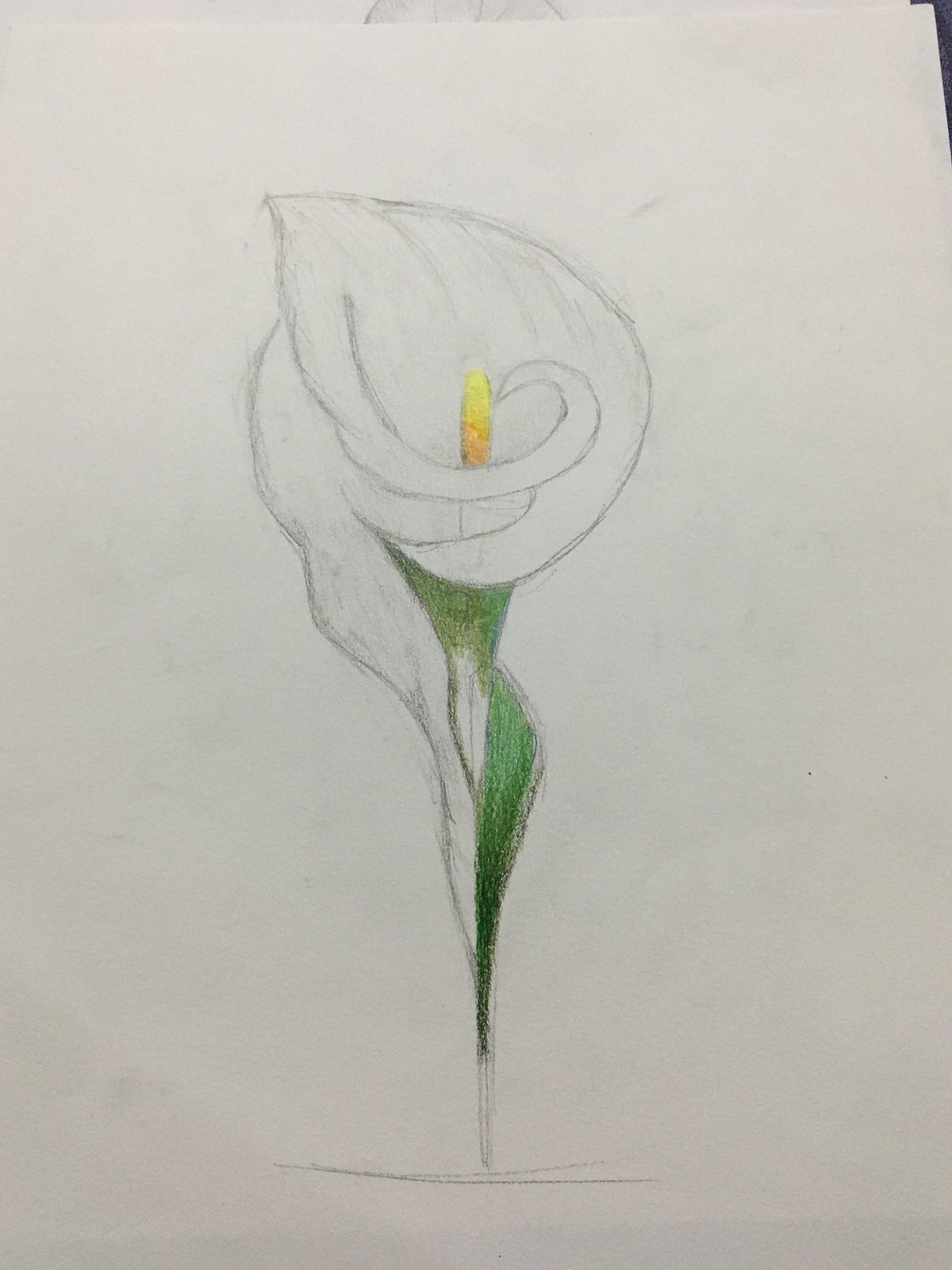A meticulously hand-drawn depiction of a calla lily flower graces this image, rendered primarily in pencil. The delicate outlines of the petals showcase intricate detailing, characterized by soft, light gray shading. The stamen at the center of the flower is vividly highlighted in a bright yellow hue, offering a striking contrast to the otherwise monochrome illustration. Additionally, the lower segment of the plant, encompassing the stem and base of the leaf, is animated with a lush green colored pencil, adding a touch of vibrancy. The drawing, captured in a photograph of a piece of paper, exhibits the artist's careful attention to both form and color.